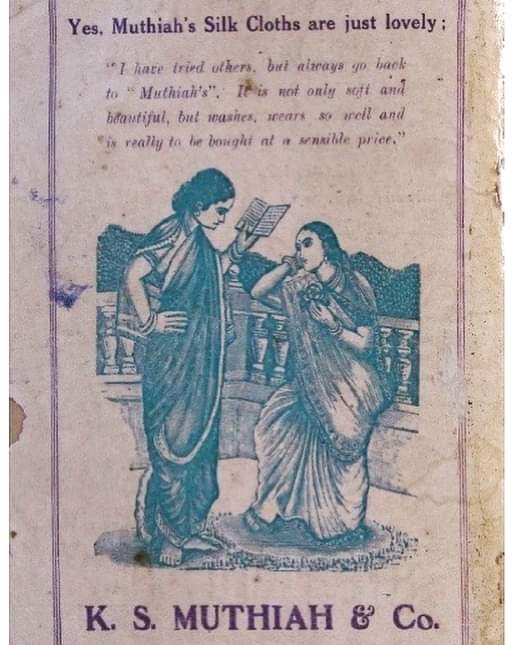The image appears to be an aged, stained page from an old book, with a brownish-white background covered in spotting indicative of its antiquity. Central to the page is a black-and-white illustration of two women dressed in Indian robes, or saris, suggesting an old-time setting on a luxurious, palatial balcony. One woman, standing with a book in hand and her other hand on her hip, faces the other woman, who is seated at the edge of the ornate patio, listening intently. Above them, a partly faded caption extols the virtues of Muteya's silk cloths, noting their softness, beauty, durability, and sensible pricing. Additional text at the bottom confirms the scene as an advertisement, mentioning "K.S. Muteya and Co." The font of the text appears in a dark purple hue, further adding to the vintage feel of the illustration.